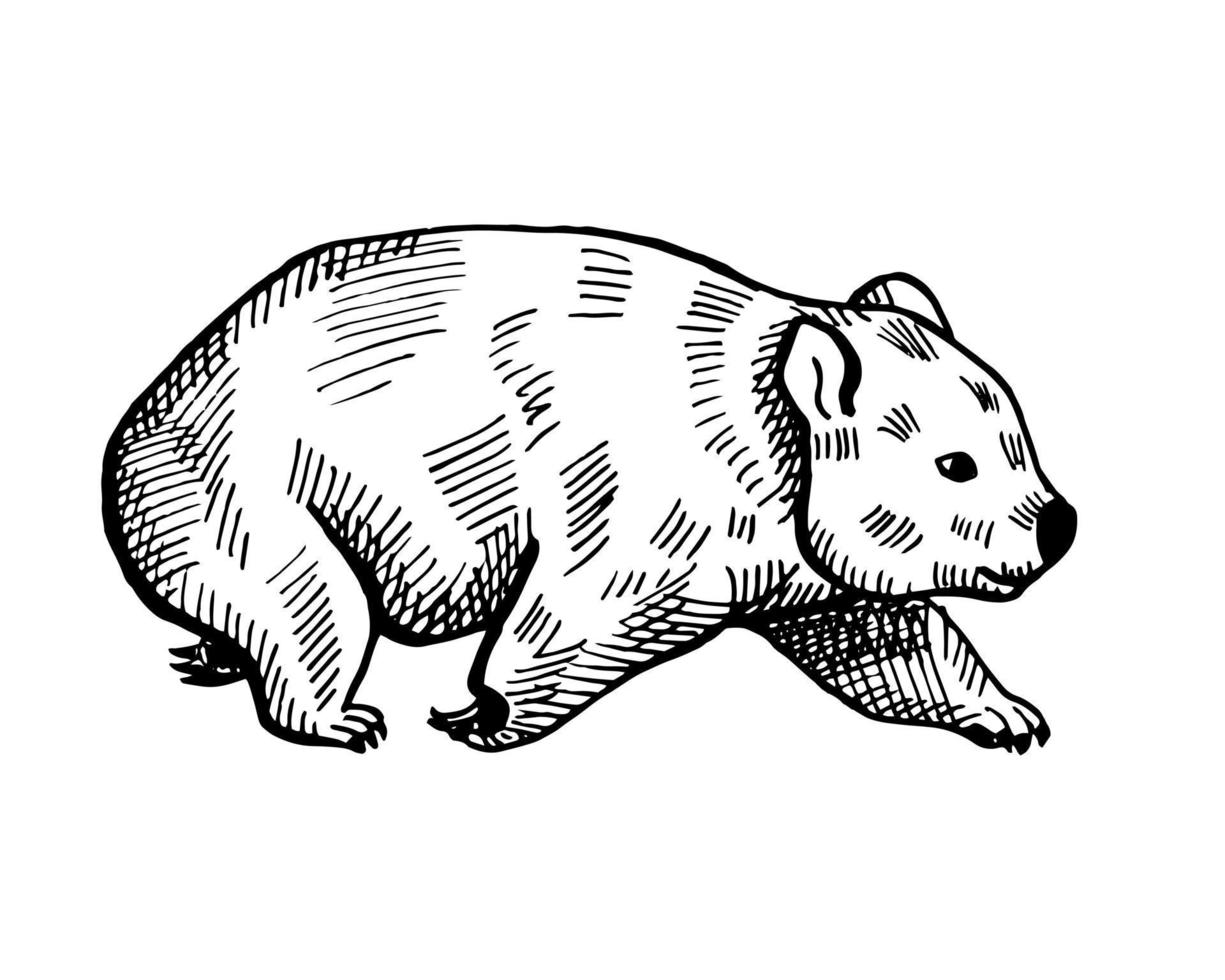This is a black and white illustration of a koala bear depicted in a side profile, facing right. The drawing is characterized by detailed black outlines against a white background. The koala is shown mid-walk, with its left front paw extended forward and its right front paw tucked underneath it. The left hind leg is positioned forward while the right hind leg is extended backward. The koala's fur is illustrated with short black lines and hash marks, especially dense and dark on its back and legs, varying in groupings such as sets of five, four, and six. The creature’s facial features include outlined black ears, a white and black eye, a circular black nose, and a simple black line mouth. The claws on each of its paws are distinctly drawn in black, with the sharpness particularly visible on the extended left front paw.